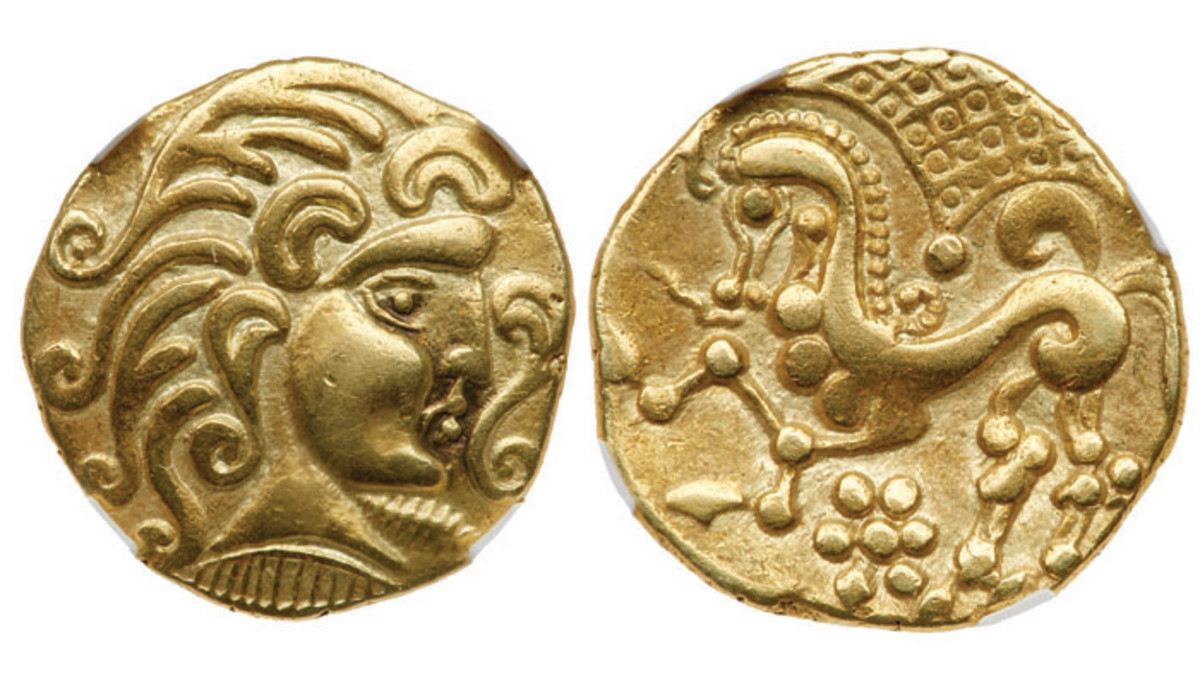Displayed are two ancient medallions with an aged, golden hue. Their shapes are roughly circular but notably uneven around the edges, giving them a distinct, handcrafted appearance. The first medallion features an intricately carved figure of a woman with long, flowing hair and a prominent, embellished collar, showcasing exceptional detail. The second medallion depicts a slender horse, its four legs adorned with small, circular accents. A delicate six-petal flower is etched at the bottom center, adding to the medallions' intricate artistry and historic charm.